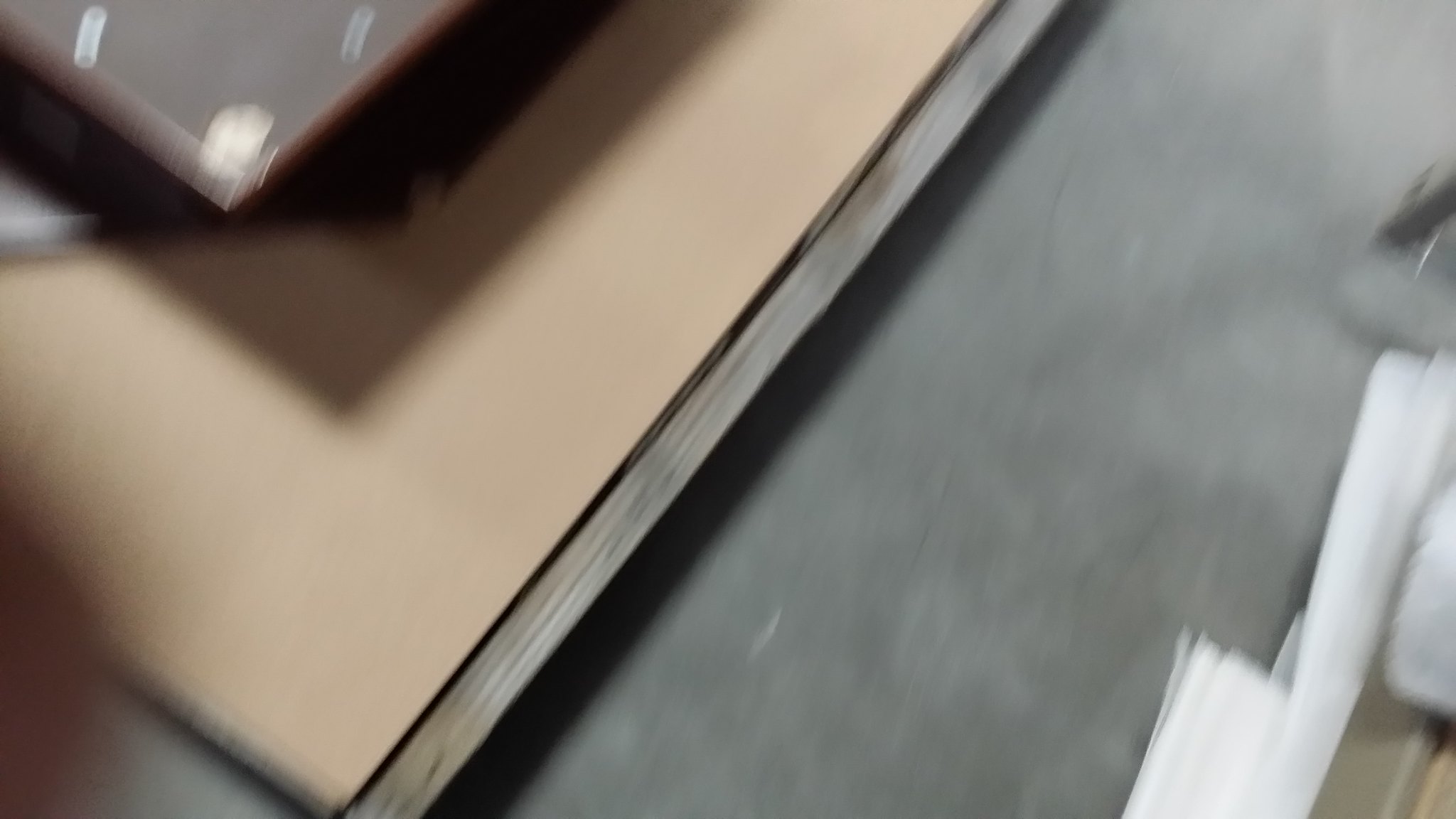On a sleek gray desk, there sits a distinctly dark reddish-brown box with white circular designs that presumably contain some text, though it is too small to discern. The box rests atop a piece of brown paper, adding a layer of contrast against the desk's surface. To the right of the box, there appears to be a white object, possibly a stack of paper or another white item, providing an additional element to the desktop arrangement.